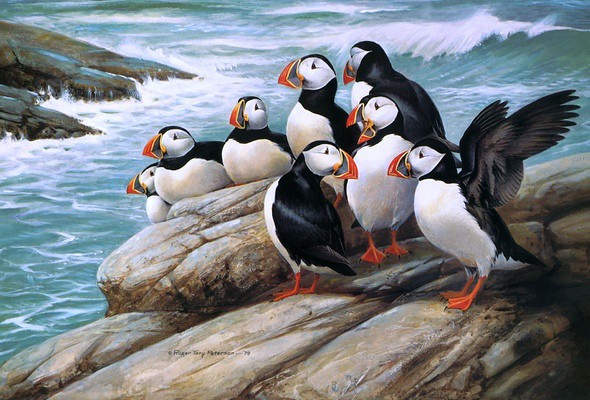The image is a colorful drawing of eight seabirds, resembling penguins but with distinct features, all gathered on a rocky outcrop in front of a choppy ocean. The birds have striking black wings and backs, white underbodies, and a unique black and white head pattern – a white triangular shape encasing their eyes. The large, prominent beaks are predominantly red with yellow lines and black near the face, and they sport bright orange webbed feet. In the backdrop, waves crash against several distant rocks, adding to the oceanic setting. Some birds are perched upright, one with wings spread, while others are calmly resting. The rocky foreground is a mix of gray and yellow hues. The image also features small text likely indicating the artist's name, "Roger Terry Peterson," along with a possible date at the bottom.